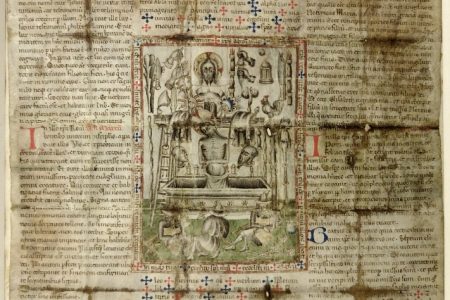The image showcases an ancient illuminated manuscript with a central illustration that appears to depict a biblical scene, featuring a haloed figure resembling a saint or possibly Jesus. Surrounding this central figure are several other people, some of whom are seated on the ground, one possibly in a tub, and another in a box with their head tilted. The illustration is detailed yet partially obscured, making specific elements difficult to discern, though a rooster and some sort of vessel or fountain are faintly visible beneath it.

The manuscript itself is handwritten in exquisite script that appears to be an old European style, likely pre-medieval or early medieval, and features gold and black ink, though some of the black ink has faded to brown. The text is interspersed with enlarged initial letters, including notable blue and red ones, such as two red "T"s and a large blue "B". Decorative elements like Maltese crosses adorn the text in blue and red, adding to the ornate nature of the manuscript. The paper shows signs of considerable age, with visible folds and dark stains along the creases, suggesting it has been handled and preserved over many years. Despite the wear and tear, the manuscript remains a striking example of historical religious art and literature.